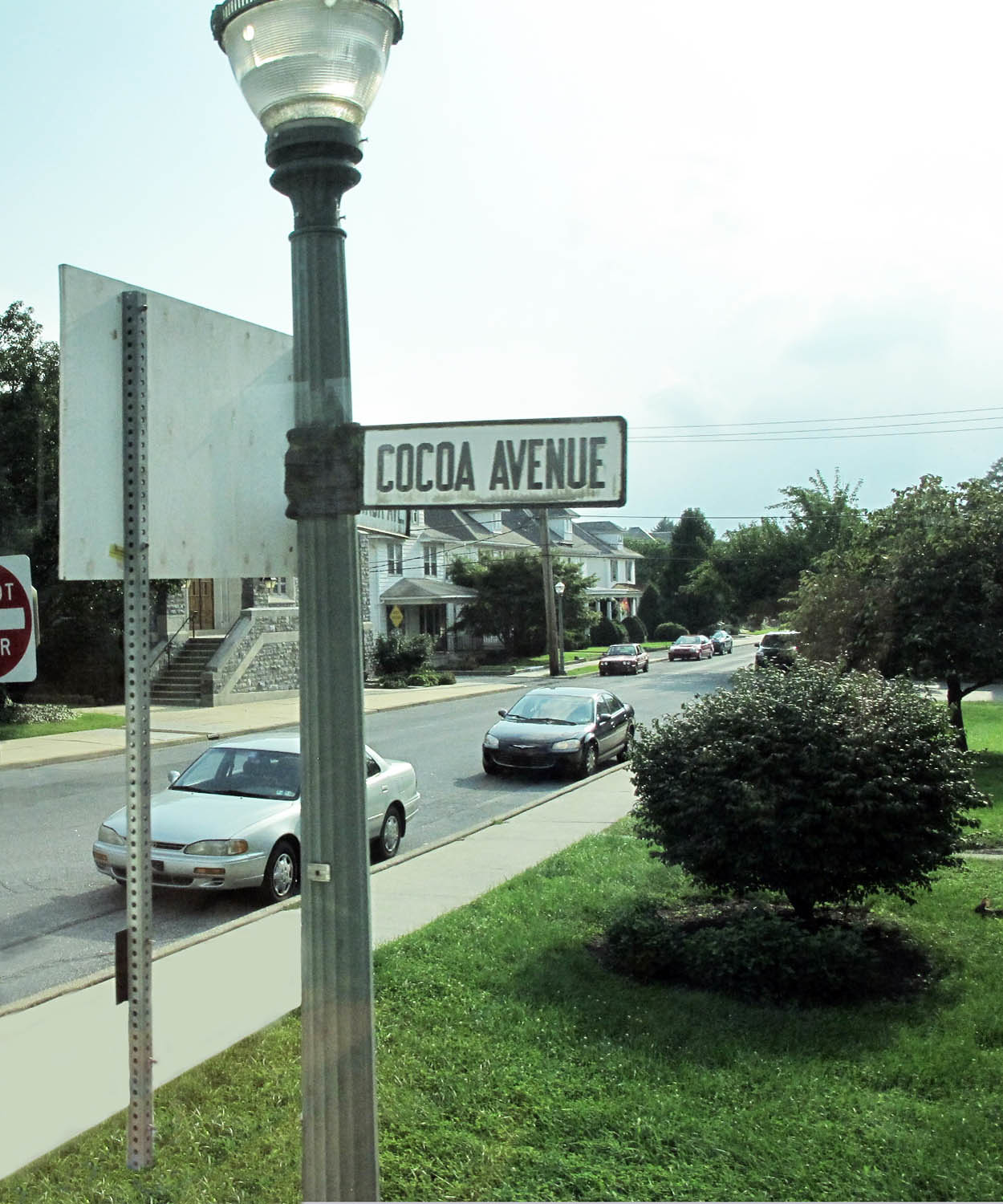In this daytime scene, a pristine white street sign with gray lettering reads "Cocoa Avenue," attached to a tall, steel, old-fashioned streetlight pole that likely functions as a gas lamp at night. The background reveals a clear blue sky dotted with white clouds and a row of trees with lush green foliage. The street scene includes several Victorian-style houses, each with steps leading up to their front porches, bordered by manicured sidewalks and lawns. A mix of wild, bushy shrubs and bright green trees line the street, which boasts smooth pavement. Multiple cars are parked along both curbsides, with a clearly visible red and white "Do Not Enter" sign on the left side of the scene. Further in the background, apartment buildings and additional trees can be seen, adding depth to the quaint residential street.